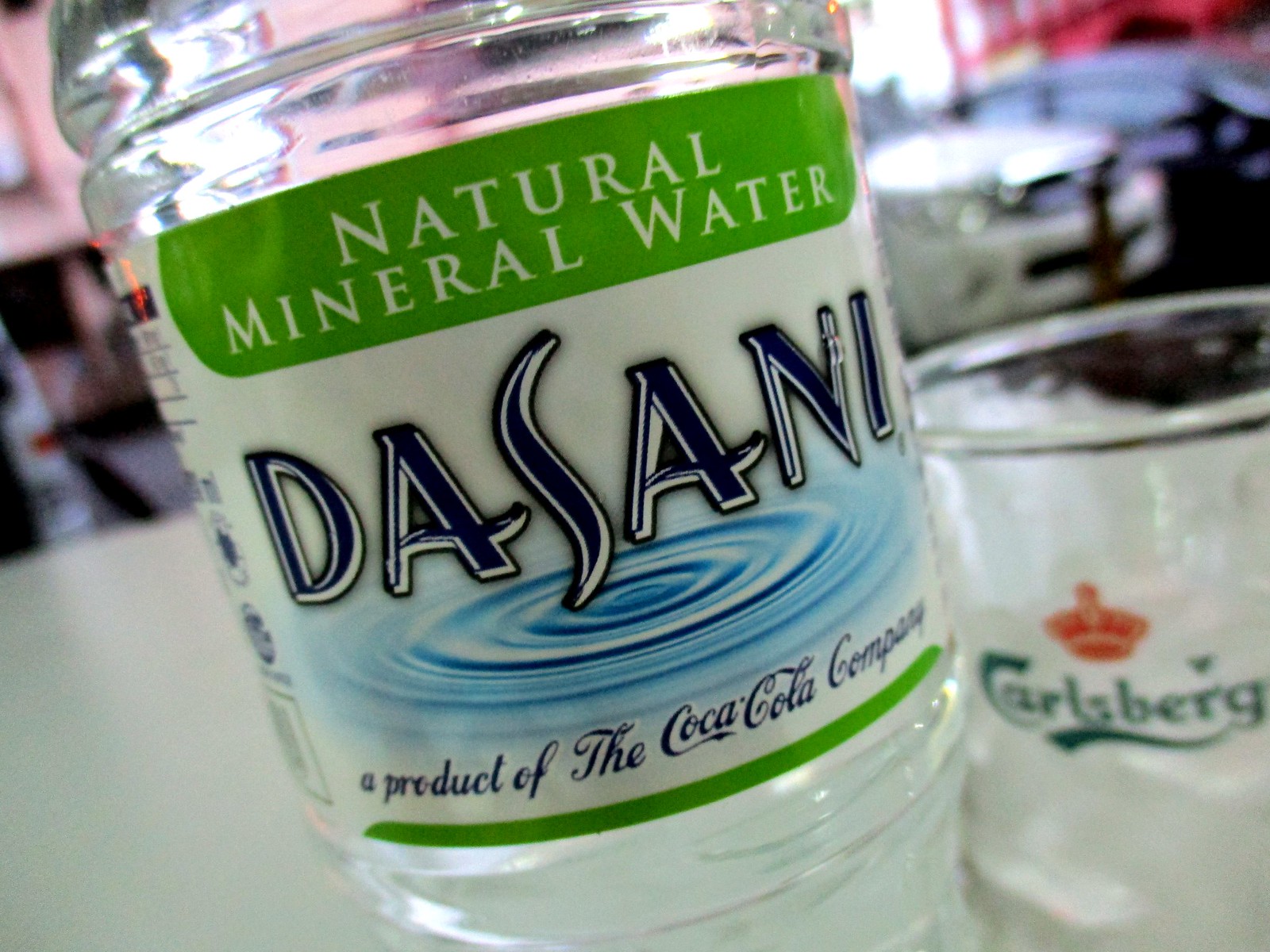The image captures a close-up, tilted view of a clear, half-full Dasani water bottle. Prominently displayed on the green label in white text is "Natural Mineral Water," with "Dasani" in bold blue lettering below it. Further down, an artistic circular ripple pattern reminiscent of a water droplet is visible, symbolizing purity and freshness. Beneath this pattern, in delicate blue cursive, the text reads "a product of the Coca-Cola Company." To the right of the water bottle is an out-of-focus glass featuring a distinctive red crown and the word "Carlsberg" below it in green letters, subtly underlined. The background is blurred, but some cars can be discerned, adding context to the setting. Overall, the sharp focus on the water bottle's label contrasts with the indistinct surroundings, drawing attention to the product's branding and details.